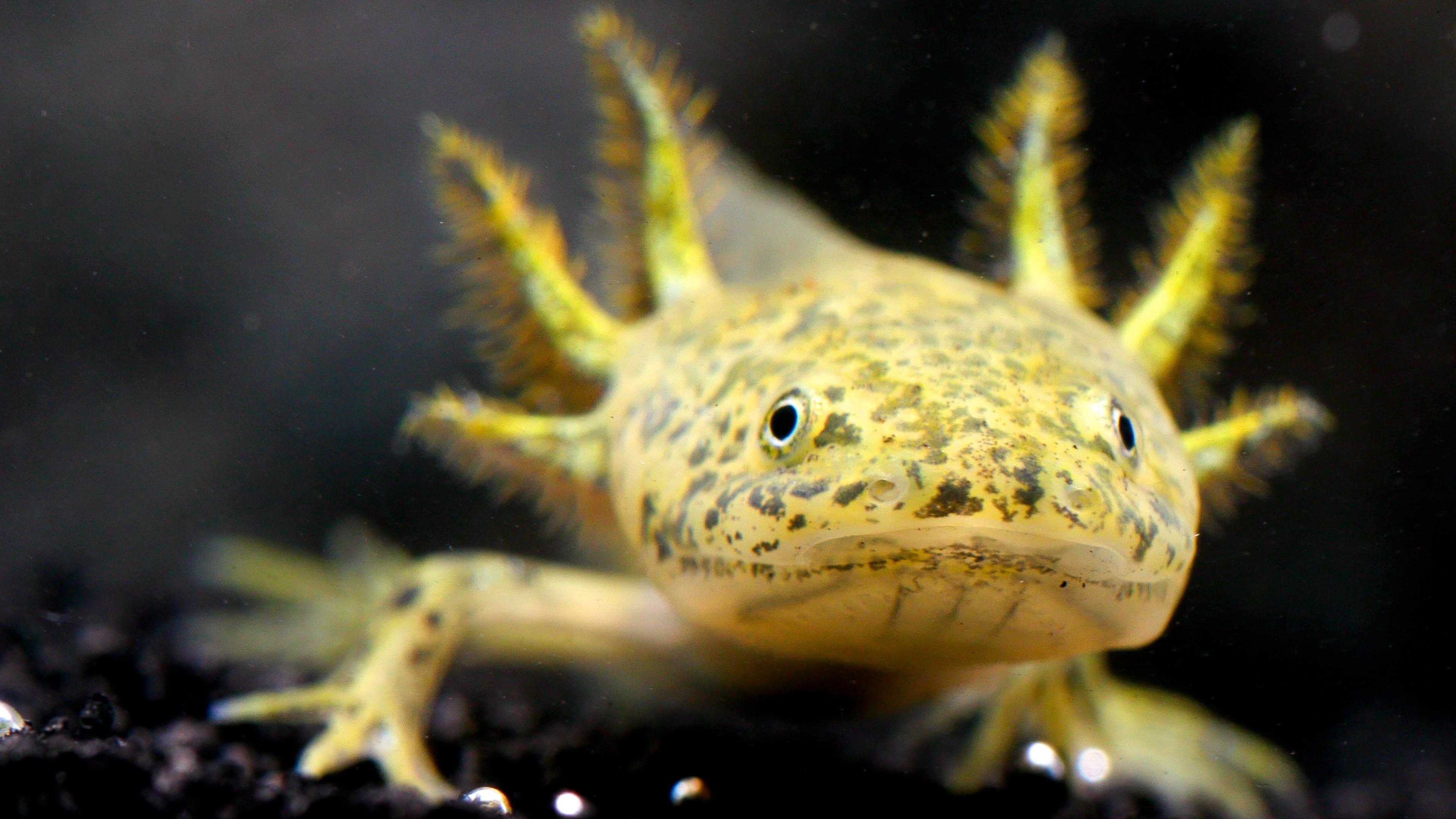This detailed underwater image features a striking close-up of a yellow salamander-like creature resting on a dark, gravelly substrate. The creature is adorned with blackish-green mottled freckles across its face, complementing its vivid yellow body and legs. Notably, it has three pointed, gill-like spikes on each side of its rounded, snake-like head, which culminates in two small black eyes with white irises. The salamander appears to be looking directly at the camera with a closed mouth, set against a predominantly black background with a hint of gray in the upper left corner. The scene is reminiscent of a fish tank environment, suggesting a controlled aquatic habitat.